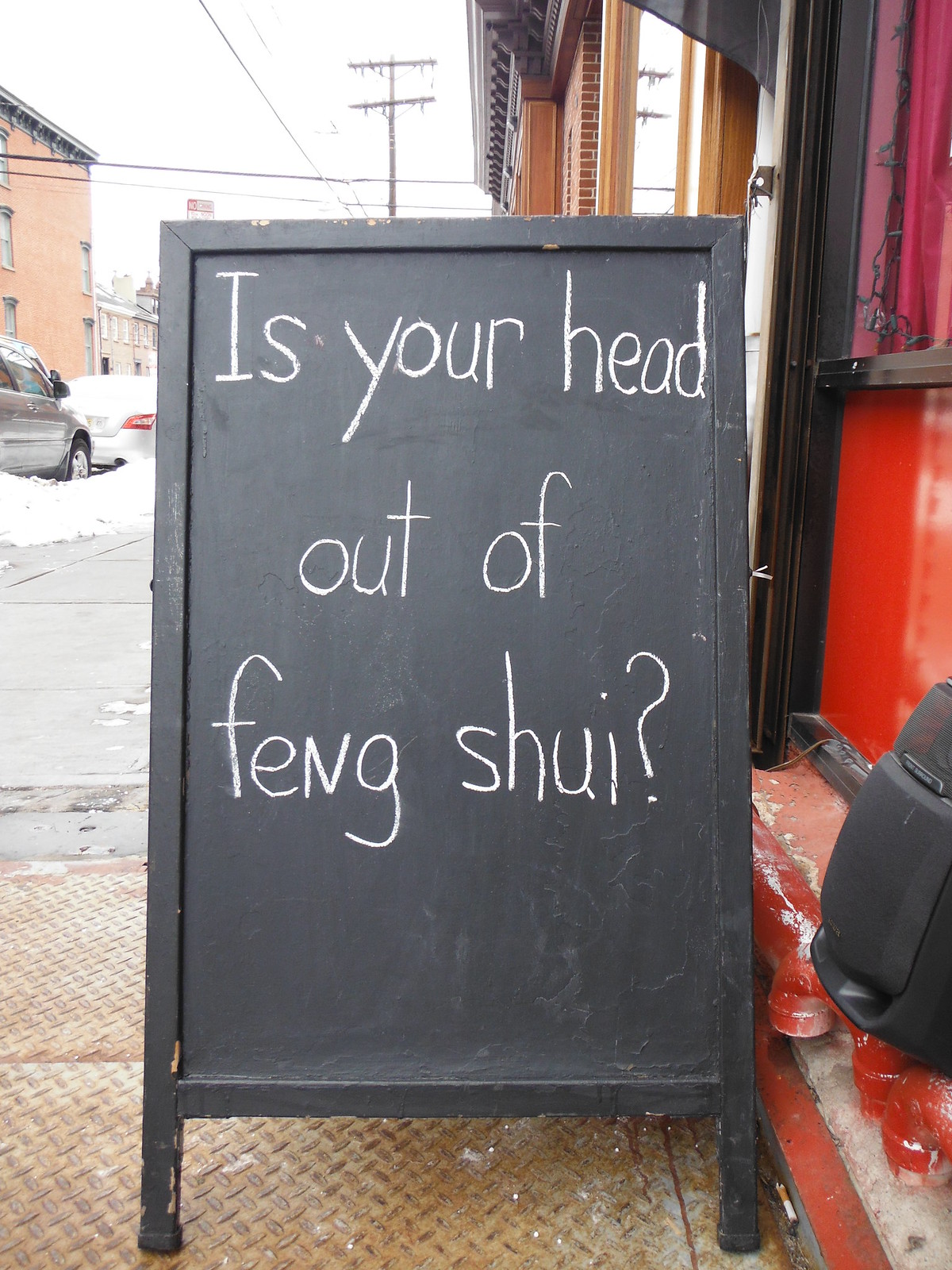In front of a red building on a brown checkered sidewalk stands an A-framed chalkboard sign with white handwritten text that reads, "Is your head out of feng shui?" To the right of the sign, there is a backpack, and behind it lies a layer of snow. The scene includes various additional details: a gray SUV is parked facing away from the viewer, a brown building neighbors the red one, and a utility pole can be seen in the upper part of the image. To the left of the blackboard, there is a brick apartment house, and two more cars are parked along the sidewalk. The black sign stands above a ground grate, near what appears to be the door of the red building.